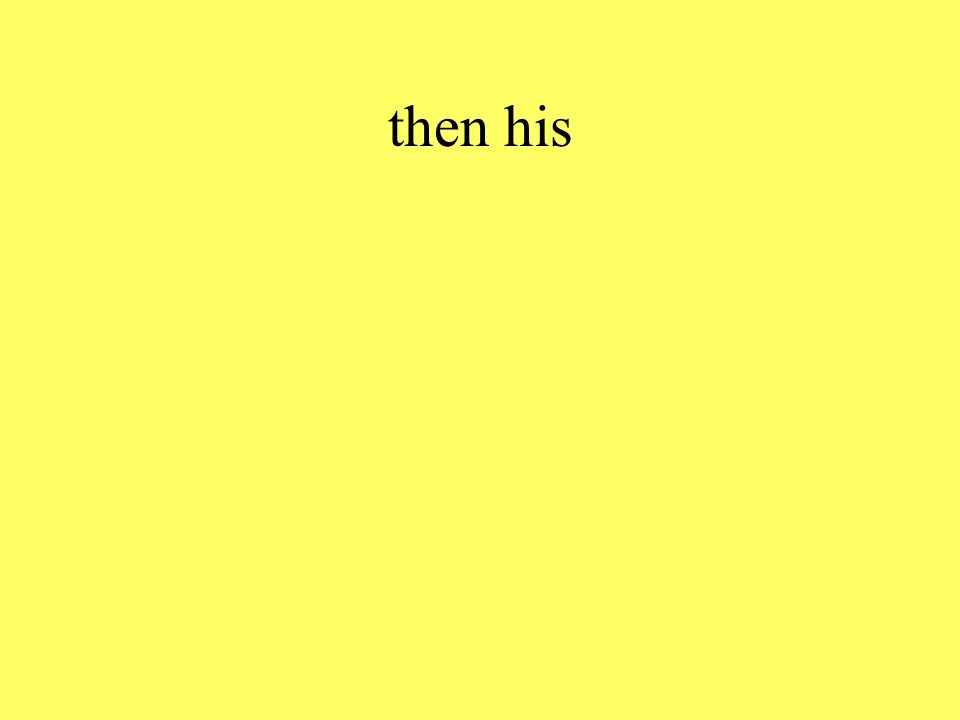The image showcases a large, light yellow square with a minimalist design. At the top center of the square are the words "then his," written in black, lowercase letters in a regular type font. There are no other elements present in the image, giving it a very modern and simplistic aesthetic.